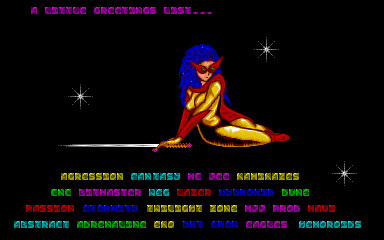This image appears to be a screen capture from a video game, presented in a landscape orientation within a rectangular frame. The background is predominantly black, contrasted sharply by various bright neon colors that create a dynamic and visually striking effect. At the top of the image, there is text that reads "a little greetings list..." adding a sense of introduction.

In the center of the composition, a female character is prominently displayed. She is seated on her right hip, leaning towards her right side, and is holding a sword that is parallel to the ground, suggesting readiness and vigilance. Her positioning and the weapon suggest that she may be a warrior or a heroine within the game's narrative.

To add to the mystique, three star-like lights radiate around the character, enhancing the ethereal and fantastical atmosphere of the image. Directly below the character, a list of words is displayed, each likely representing different elements or factions within the game. These include: "Aggression," "Fantasy," "MC," "Kamikazes," "Bizmaster," among others, indicating a diverse and multifaceted game world.

Overall, the image combines a rich palette of neon hues, intriguing text elements, and a central figure that captivates the viewer, offering a glimpse into an adventurous and vibrant game universe.